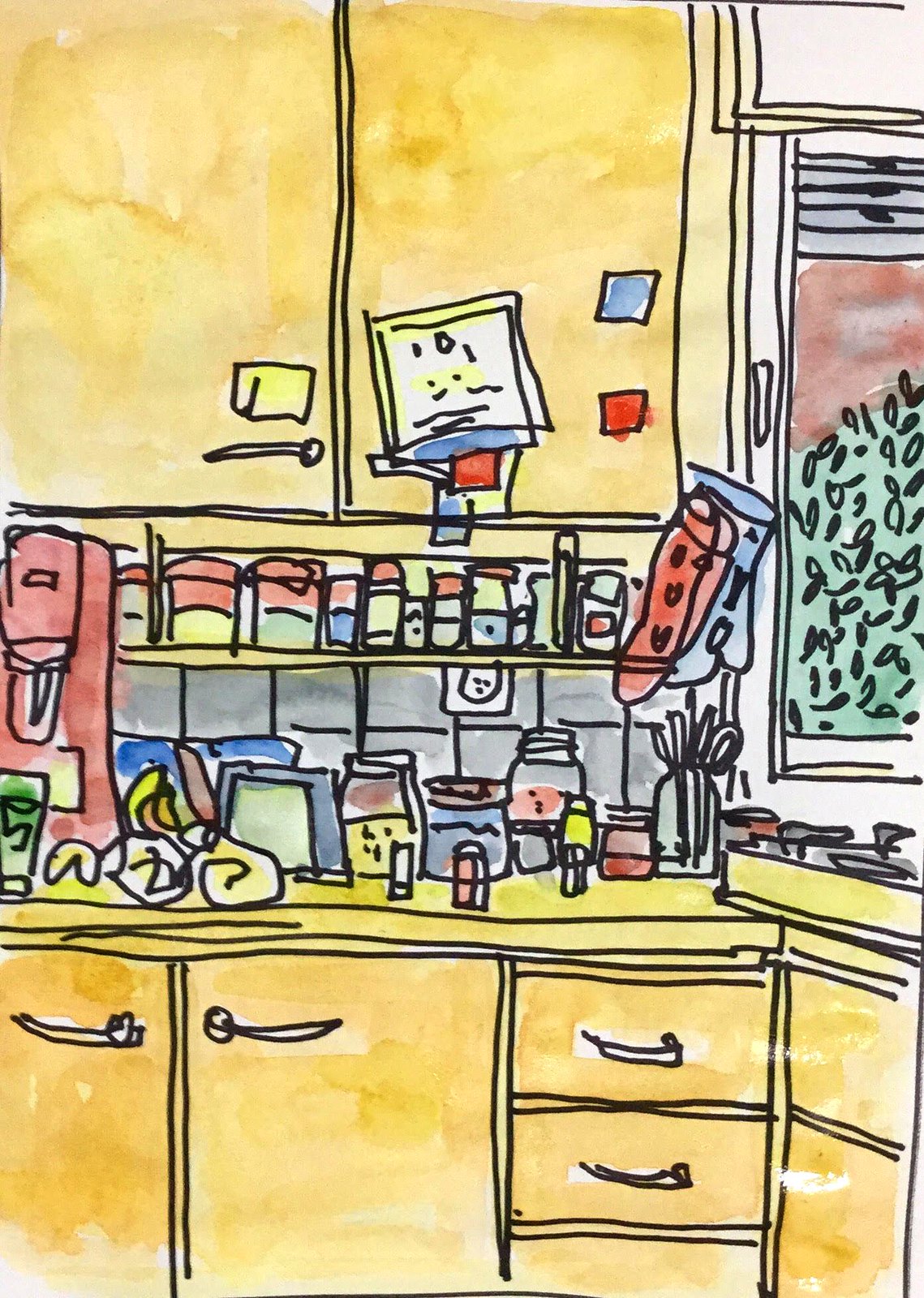The artwork depicted in this image resembles a charming illustration from a children's book, characterized by its whimsical and vibrant style. The scene is set in a cozy kitchen, meticulously outlined with black ink and vividly brought to life with watercolor paints. The kitchen space features several cabinets and drawers, their simple yet detailed design adding to the homely atmosphere.

On the countertop, a collection of jars and a prominent red mixer catch the eye with their bright colors and fine detailing. Above the countertop, the shelves and cabinets hold various kitchen essentials, including a small rack beneath them that neatly displays an array of spice cans.

To the right of the image, a window with its shades pulled up offers a glimpse of the world outside. Through the glass, a lush scene of green trees and bushes is beautifully painted, adding a touch of nature to the cozy, indoor setting. The overall composition blends the everyday charm of a kitchen with the playful, imaginative touch of a storybook illustration.